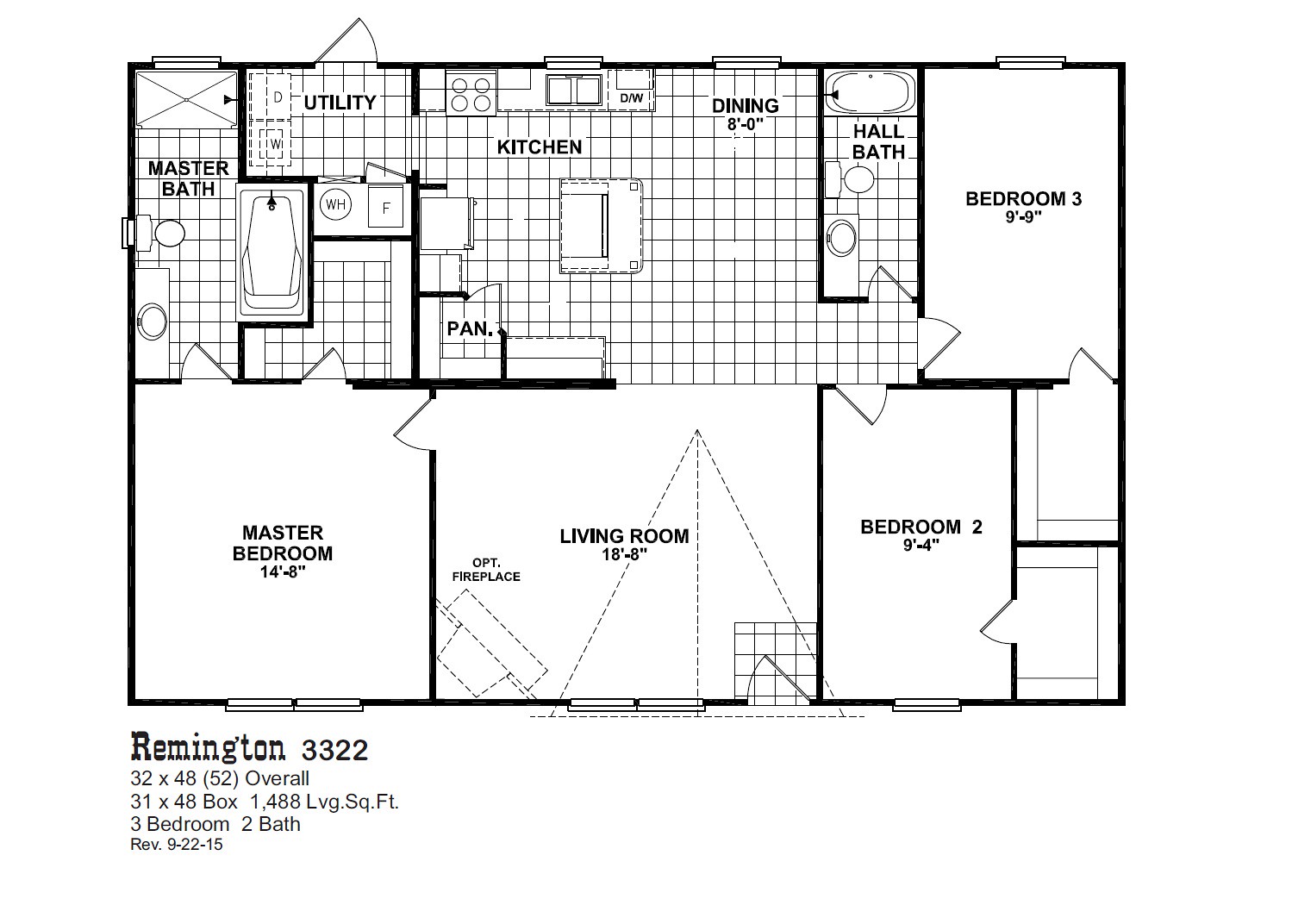This image displays the detailed floor plan of the Remington model, identified by the label in the bottom left-hand corner. The Remington floor plan is captioned "Remington 3 3 2 2" with accompanying detailed measurements, noting a revision date of September 22, 2015. This plan outlines a three-bedroom, two-bathroom residence featuring dimensions of 32 by 48 feet and an overall length of 52 feet, resulting in 1,488 square feet of living space.

In the bottom left-hand corner, the layout reveals the master bedroom, distinguished by its two windows. Moving north within the image, the master bathroom is depicted, comprising a closet, shower, toilet, and sink lined up against the wall. Adjacent to the master bathroom is an additional closet.

The master bedroom seamlessly transitions into a spacious living room measuring 18 by 8 feet. The living room is illustrated with options for a fireplace and a doorway presumed to be the main entry point. This area also includes a couple of windows adjacent to the entry door.

Central to the floor plan, the kitchen features a centrally located island, a walk-in pantry with a door, and a connected dining area. Off the kitchen is a utility room equipped with space for a washer and dryer, with an exterior door for convenient outdoor access. The kitchen layout includes allocated spaces for a stove and fridge, as well as countertops aligned along the sides, complemented by nearby windows.

Proceeding to a small adjoining nook, the plan reveals two additional bedrooms, each harboring a small attached closet. These bedrooms share a hall bathroom, which accommodates a shower-tub combination, a toilet, and a sink.